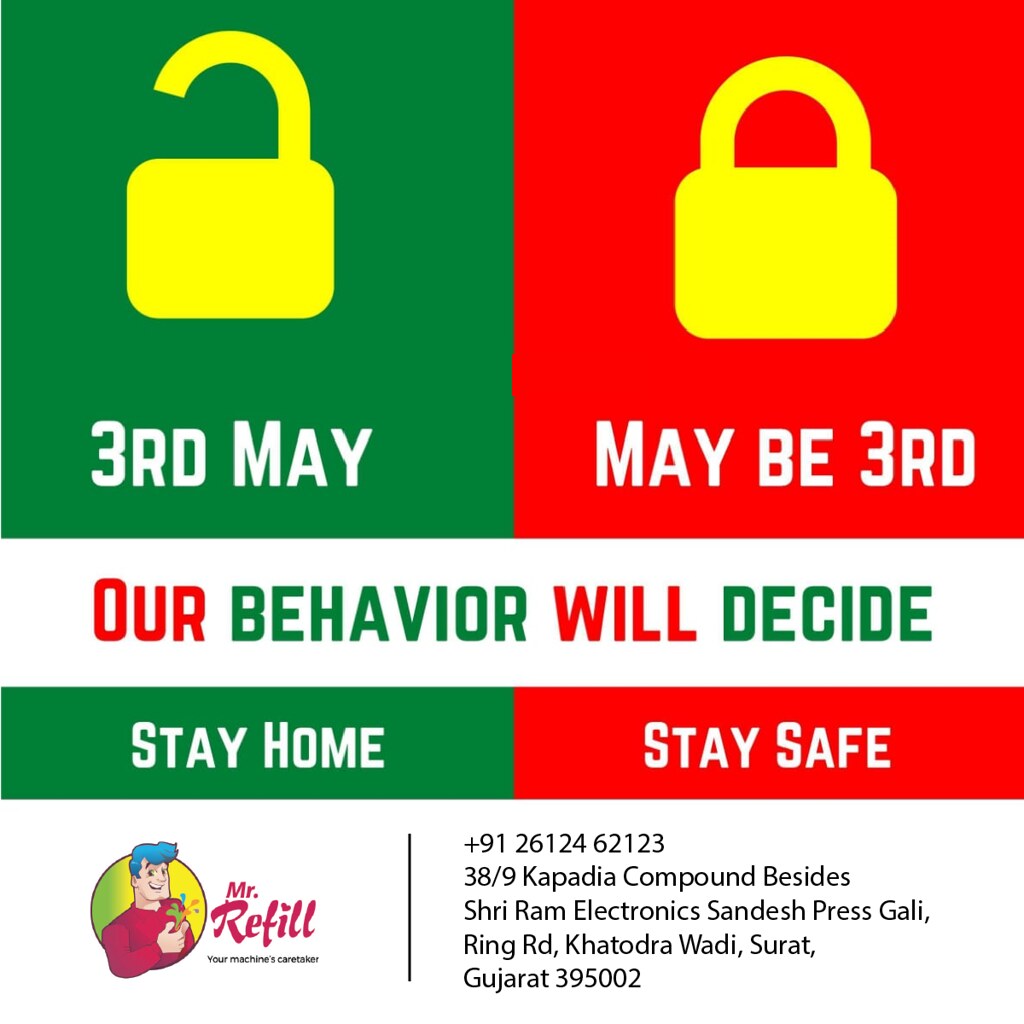The image appears to be an advertisement poster, heavily featuring bold print and a mixture of vibrant colors such as green, red, and yellow. In the top left corner, there is a green square with an unlocked yellow lock icon, accompanied by the date "3rd May" in white text below it. Right next to this, on the top right, is a red square with a locked yellow lock icon, also displaying "3rd May" in white text below. Positioned below these elements is a long horizontal white bar that contains a series of words: in red text "Hour", followed by "Behavior" in green, "Will" in red, and "Decide" in green.

Further down, occupying the left half horizontally, is a green strip with the words "Stay Home" written in white. Oppositely, on the right half, a red strip mirrors this design with "Stay Safe" also in white. Below these strips, on the left side, is a cartoon character labeled "Mr. Refill", featuring a blue-haired animated figure. Also present is the contact information: "+91-261-2462-12338/9, Capatia Compound, Besides Shree Ram Electronics, Sandesh Press Gali, Ring Road, Katorda, Wadi Falia, Surat, Gujarat, 395002". This contact block is detailed in white text, set against a background that mirrors the bold, contrasting colors of the rest of the poster.